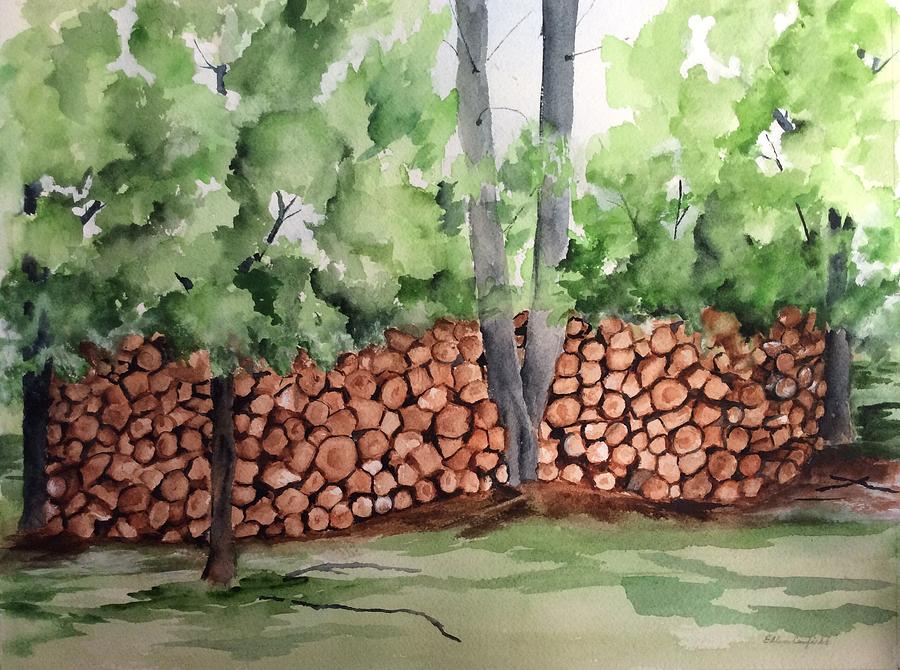This detailed watercolor painting showcases a homestead area with a focus on a neatly arranged stack of logs, prepared for winter. The logs vary, with some split by an axe and others just stacked, forming a slightly curved rectangular formation around a central tree. This tree, splitting into two trunks a few feet off the ground, is painted in dark gray, with visible dirt around its base. Surrounding this stack are four leafy trees, with one very tall tree and several shorter, foliage-rich companions. The leaves display a spectrum of greens - dark, light, and lime, illustrating the surrounding forest environment. The ground features a blend of muted greens and beige, indicating different shades of grass and earthy ground. Above the scene stretches a cloudy, light gray sky, hinting at an overcast day.